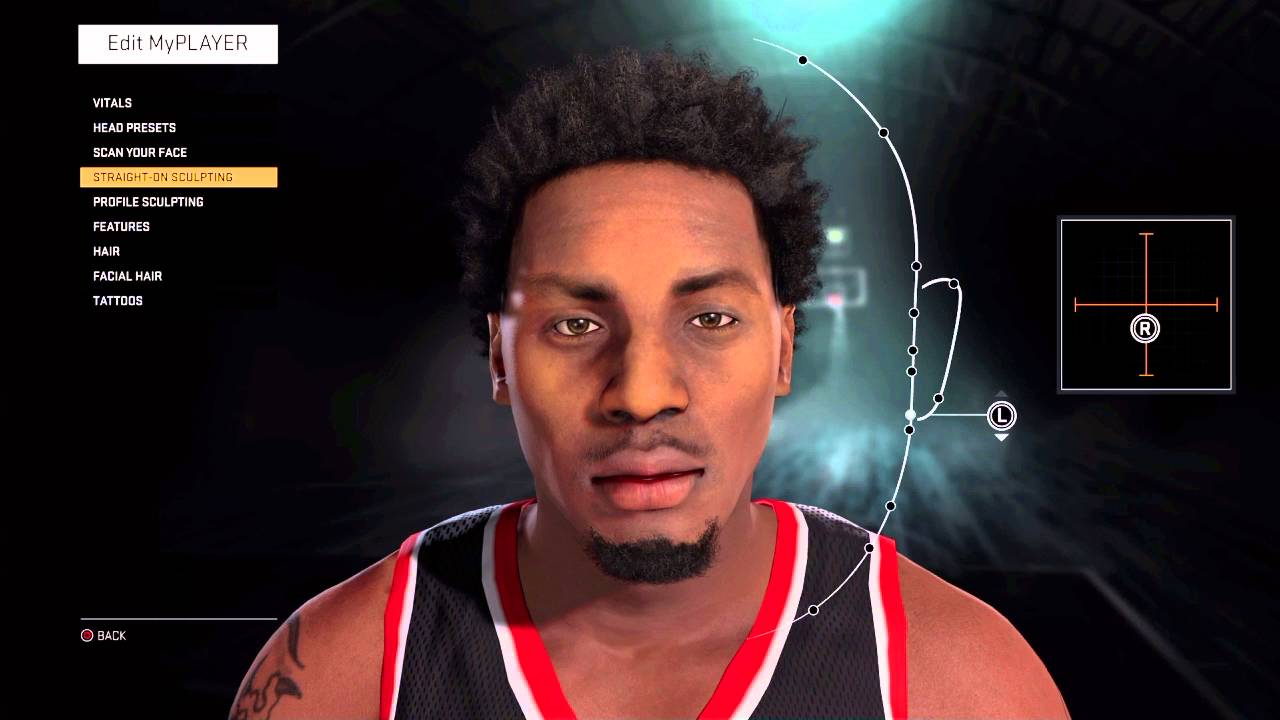An illustration of a basketball player is depicted on this online webpage, set against a predominantly black background. The image is rectangular, in a landscape orientation. Positioned in the center, the player is shown from roughly the armpits up, wearing a black sleeveless basketball uniform with red and white trim. He has darker skin and sports a fairly thick goatee complemented by a thin mustache. His hair is black and mildly afroed. The player gazes directly at the viewer with a serious expression, his lips slightly parted.

Over the player's right shoulder (to the viewer's left), the dimly lit background reveals a distant basketball hoop, faintly illuminated by a pale blue light emitting from the top, casting a glow over the court. 

In the upper left corner of the image, a white rectangle contains the text "EDIT MY PLAYER." Below it are nine selectable options in all caps white text: VITALS, HEAD PRESETS, SCAN YOUR FACE, STRAIGHT ON SCULPTING, PROFILE SCULPTING, FEATURES, HAIR, FACIAL HAIR, and TATTOOS. The fourth option, STRAIGHT ON SCULPTING, is highlighted with a yellow background and black text, indicating the current selection.

To the far right, there's a square interface element with a plus sign, showing some form of control mechanism. It features an "R" and a double white circle. Near the player’s face on the viewer's right, a semicircular bracket extends from above his head to below his chin. Attached to it is a line marked with an "L" and a double circle, suggesting additional editing functions being applied to the image.